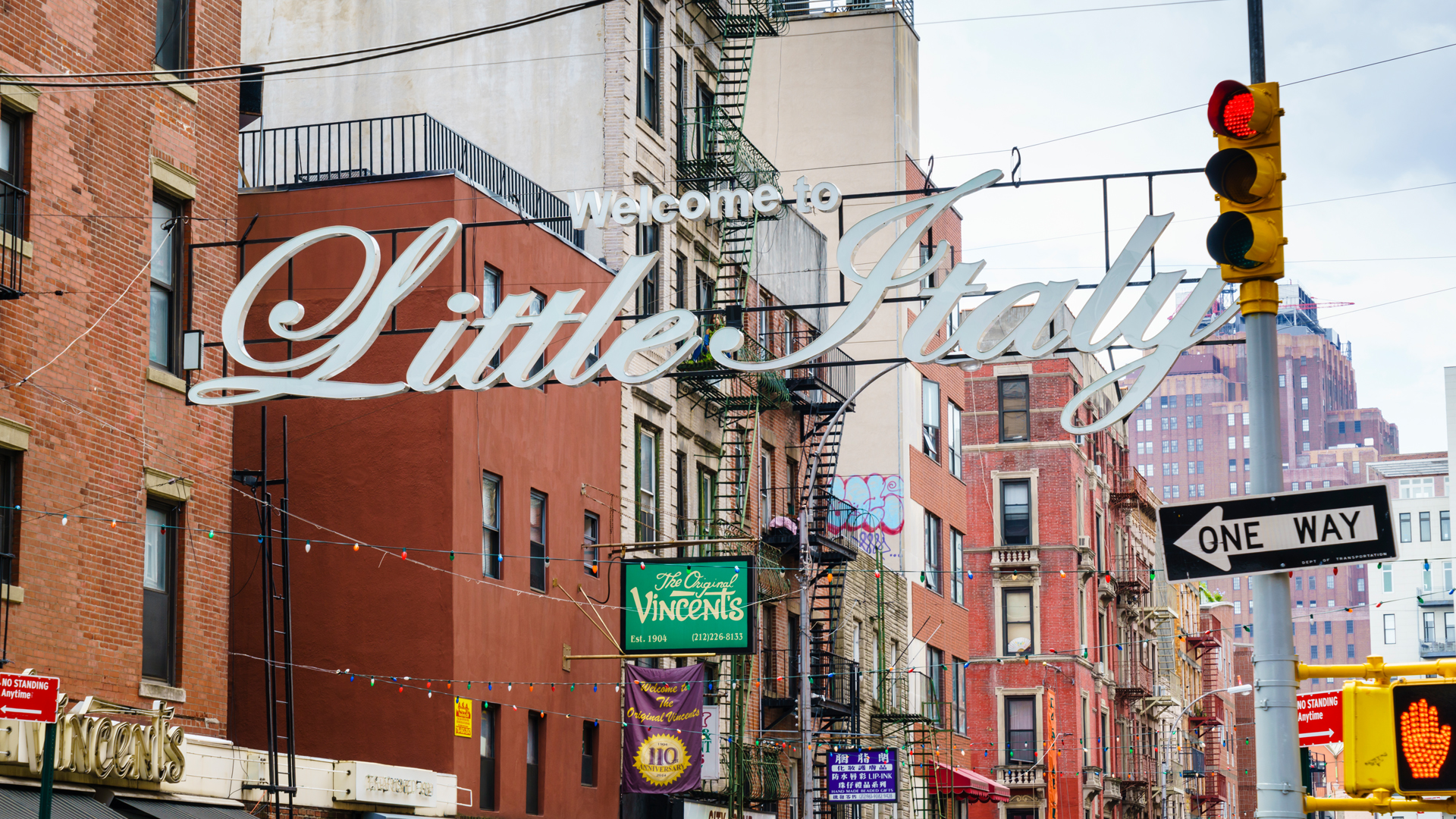The image showcases a bustling downtown cityscape marked by a prominent street sign reading "Welcome to Little Italy," with "Welcome to" in standard print and "Little Italy" in cursive font on a white, potentially illuminated material set within a black frame. Below the sign, a red traffic stoplight and a One Way sign are visible, alongside a no-walking light indicated by a yellow box with a hand symbol. The scene features multiple inhabited buildings with signs, including a notable green sign reading "The Original St. Vincent's Established 1904" and an additional purple cloth sign commemorating the 110th anniversary, likely from the year 2014 or 2024. Various billboards and graffiti add to the urban feel, with the gray sky setting a moody backdrop.